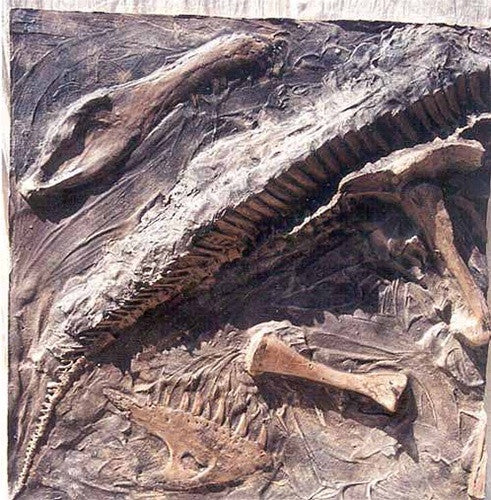The image showcases a partially excavated fossilized dinosaur embedded in a brownish, beige-tinged matrix with visible brush marks indicating the excavation process. Prominently running from the top right corner to the bottom left corner is the dinosaur's tail, which is well-defined and tapers as it extends. Adjacent to the tail in the top right is a large, pronounced leg bone. The upper jaw with visible teeth and an eye socket is positioned towards the middle, slightly on the lower side, hinting at the skull's location. Scatterings of other bones, including what appears to be another leg bone and a section of the lower jaw, are also present. The overall scene suggests an active archaeological dig, with bones standing out amidst a textured, painted fossil bed.